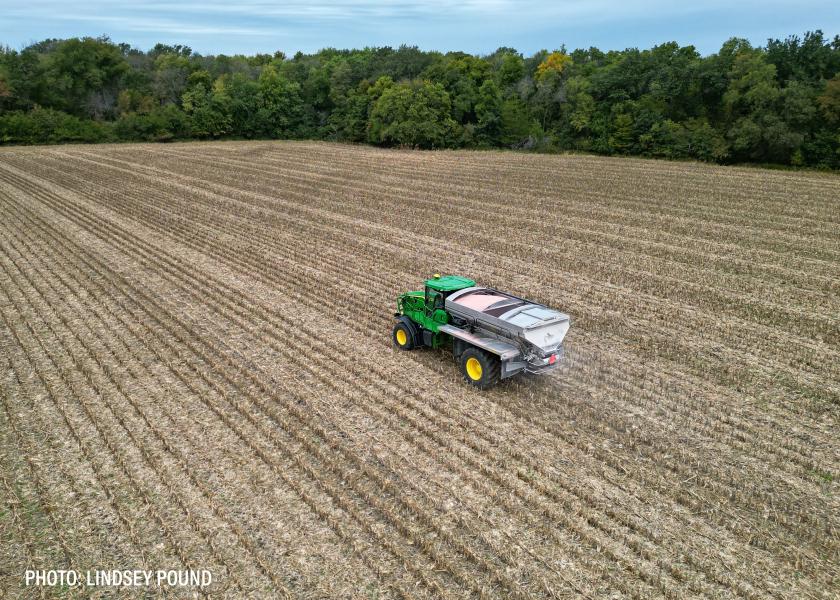In this detailed photograph by Lindsey Pound, as indicated in small white text in the bottom left corner, a vivid scene of a farm field unfolds. The field, appearing freshly plowed with its dirt surface devoid of any vegetation or grass, stretches towards the horizon, suggesting recent preparation for planting. It features undulating layers created by plowing. Dominating the center of the image is a distinctive green farm truck with conspicuous yellow wheels and large black tires; its bed is a gleaming silver, possibly a seed distributor. The backdrop showcases a line of dense, vibrant green trees, their foliage rich and healthy. Above them, a clear blue sky creates a striking contrast to the earthy tones below, capturing a serene, yet industrious rural landscape.